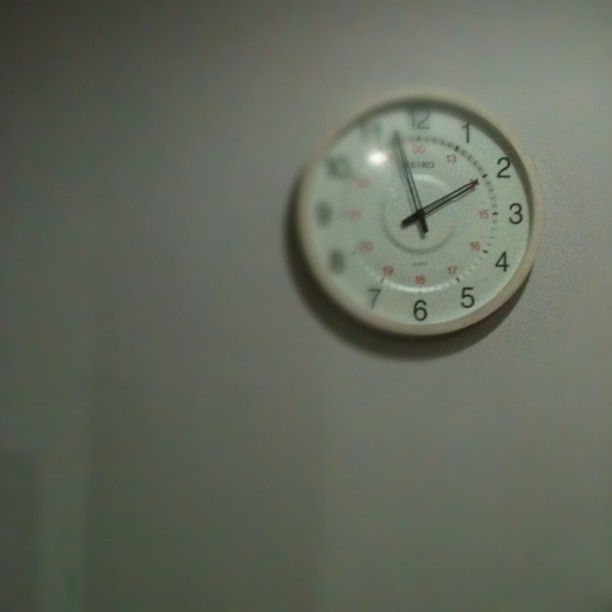This photograph showcases a simple yet somewhat blurry image of a wall clock with a beige or white plastic frame, hanging on a very light gray or white wall. The clock has a white face with bold black numbering for each hour from 1 to 12, and is branded with the label "Seiko." The minute and hour hands are black, with the hour hand pointing towards the 2, and the minute hand positioned between the 11 and the 12, indicating approximately 1:57. There is some noticeable blurring on the left side of the clock, specifically from the 8 to the 11, which might be due to light reflection or some damage. Additionally, smaller red numbers are situated inside the clock face, incrementing every hour to depict military time, starting at 13 for 1, 14 for 2, and so on.